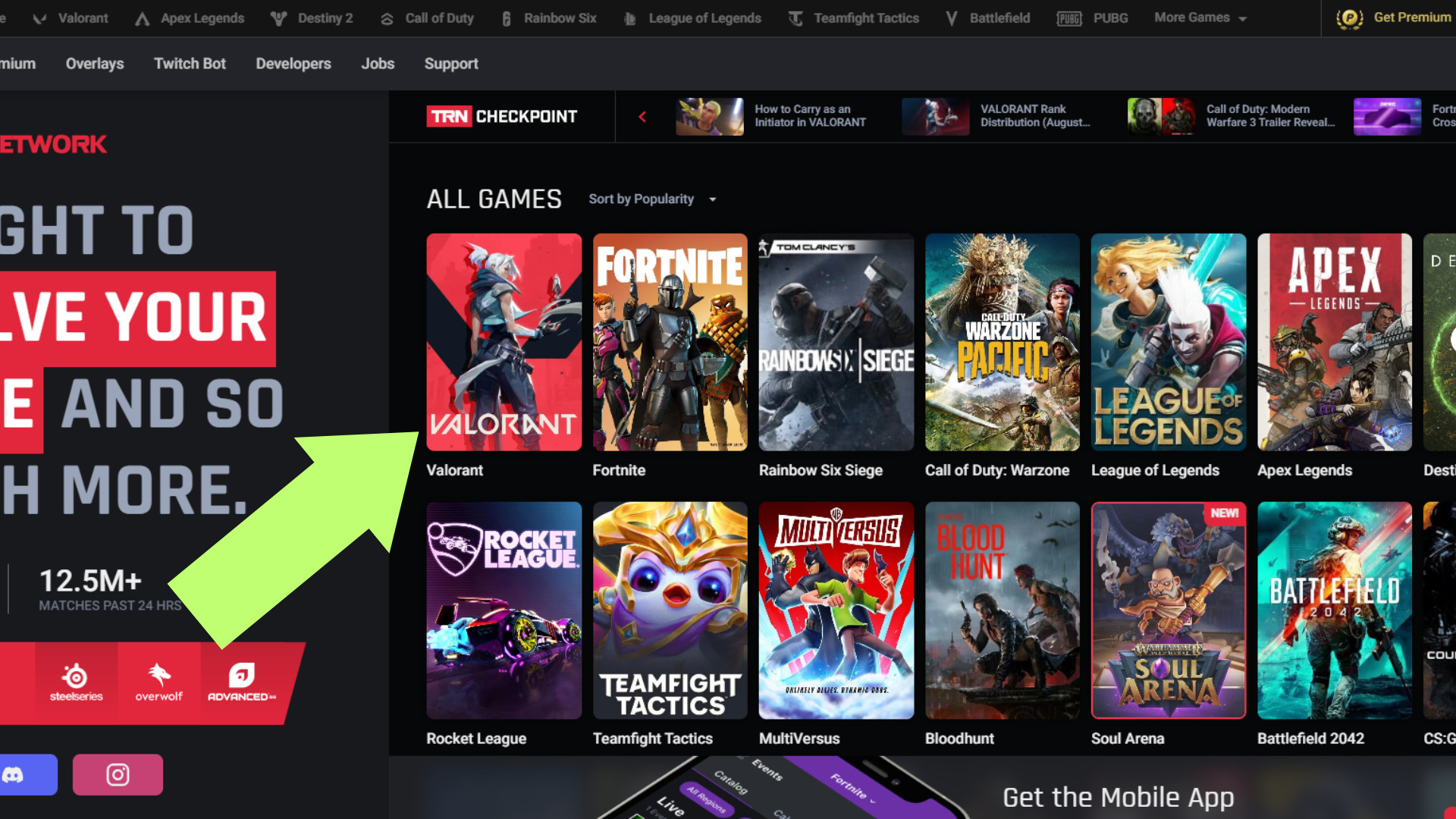The screenshot features a black background with two horizontal rows of thumbnail images, each row containing six computer game icons, positioned on the right side. The games showcased include, from top to bottom: Valorant, Fortnite, Rainbow Six Siege, Call of Duty Warzone Pacific, League of Legends, Apex Legends, Rocket League, Teamfight Tactics, MultiVersus, Blood Hunt, Soul Arena, and Battlefield 2042. Dominating the center-bottom area of the screenshot is an oblique section of a smartphone display, highlighted by a purple banner at the top reading "Fortnite," accompanied by a purple button on the left. A prominent green arrow, oriented diagonally from the bottom-left towards the top-right, points directly at the Valorant thumbnail, accentuating its position within the array of game icons.